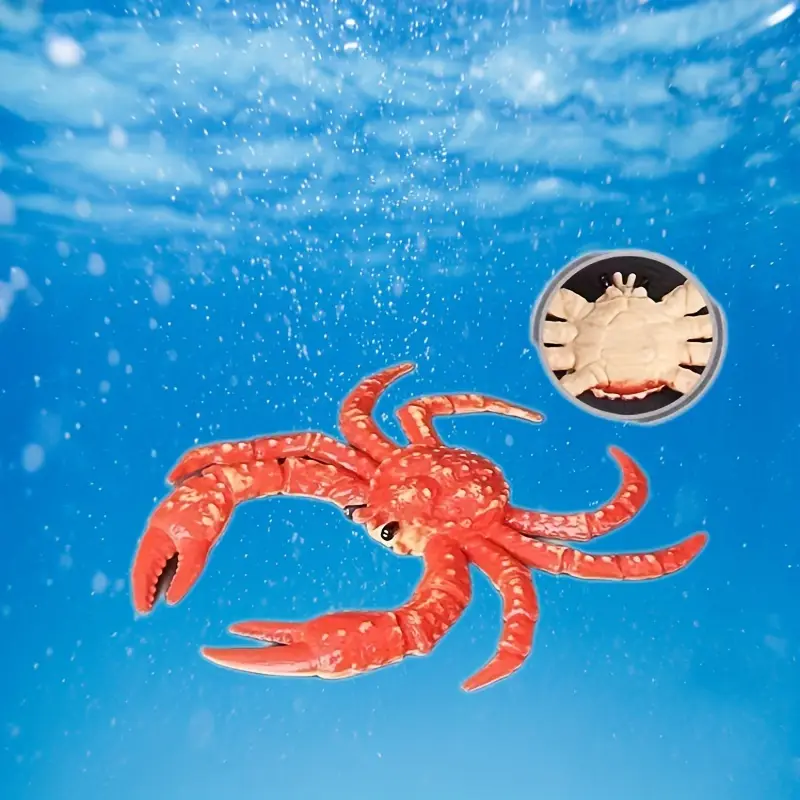The image depicts a vibrant red-orange crab, appearing almost like a painting or a toy, suspended just beneath the water's surface. The water is a light blue, illuminated by sunlight, creating a serene underwater scene. The crab, detailed with a white underside, has six legs and two prominent claws, which are slightly open. Its form is accentuated with white tips and sporadic tan or beige blotches. The crab’s beady black eyes add a lifelike touch, despite its toy-like appearance. Additionally, a circular inset highlights the crab's underside, emphasizing its white belly. Surrounding the crab are small white bubbles rising to the surface, adding to the ethereal, artistic quality of the image.